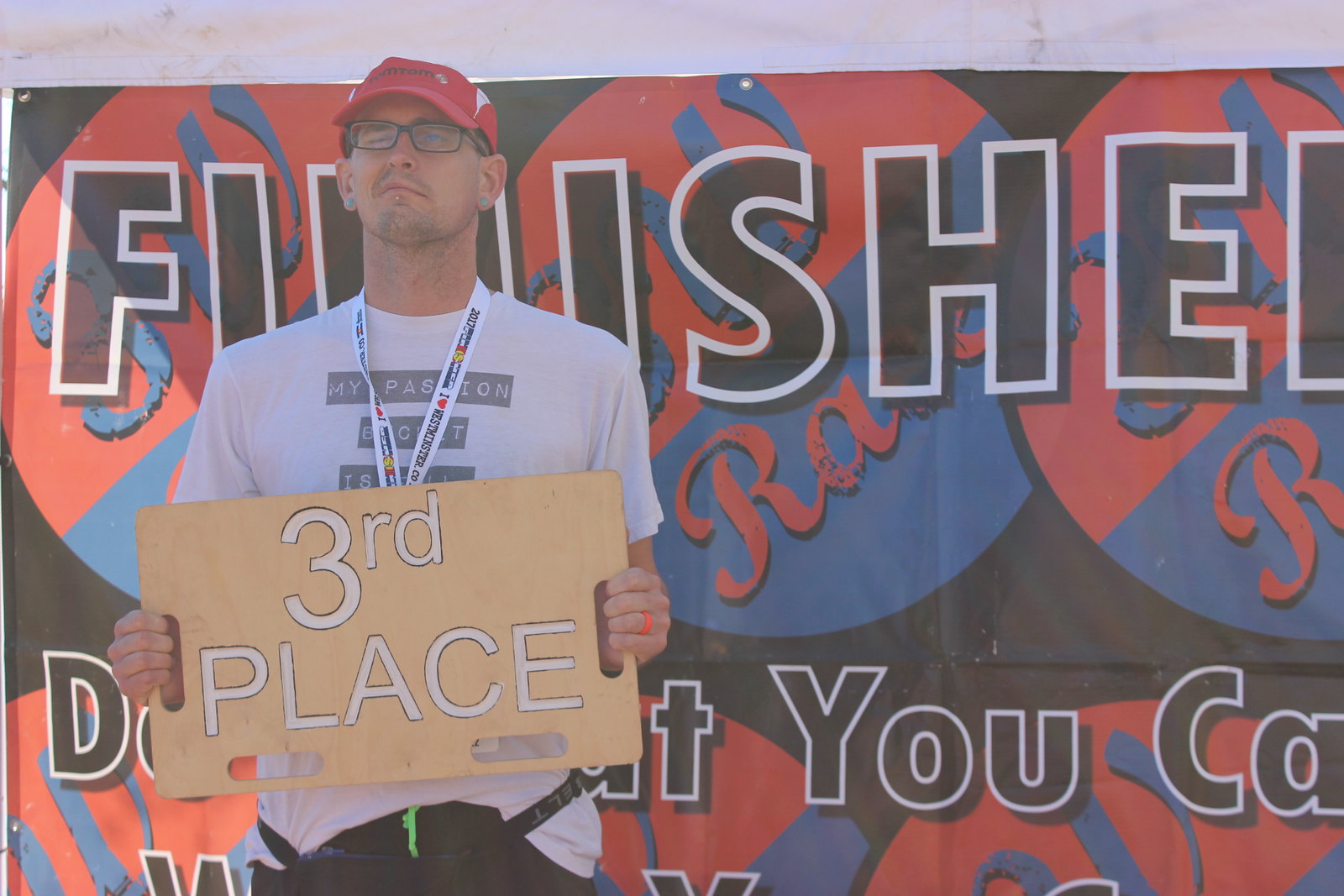This detailed landscape-style photo captures a relatively young gentleman standing to the left side of the frame. He is holding a third place sign, conveying his participation in a race or marathon, as hinted by the large, partially obscured banner behind him that reads "FINISHED." The man, seemingly in his mid-20s, wears a red baseball cap, black glasses, and a white shirt with unreadable text. Accessorized with a green earplug, a red silicone wedding band, and a fanny pack around his waist, he projects an active lifestyle.

Around his neck, he sports a lanyard, likely holding a medal, although the actual medal is hidden by the third place sign. His facial expression—a mix between a smirk and a gnarling look—does not outwardly display happiness. The banner behind him features black letters outlined in white and includes a red and blue circle with additional, unreadable text. The overall clutter and position of elements make parts of the scene difficult to discern, but it is clear that this image captures the complex emotions of achieving third place in a competitive event.